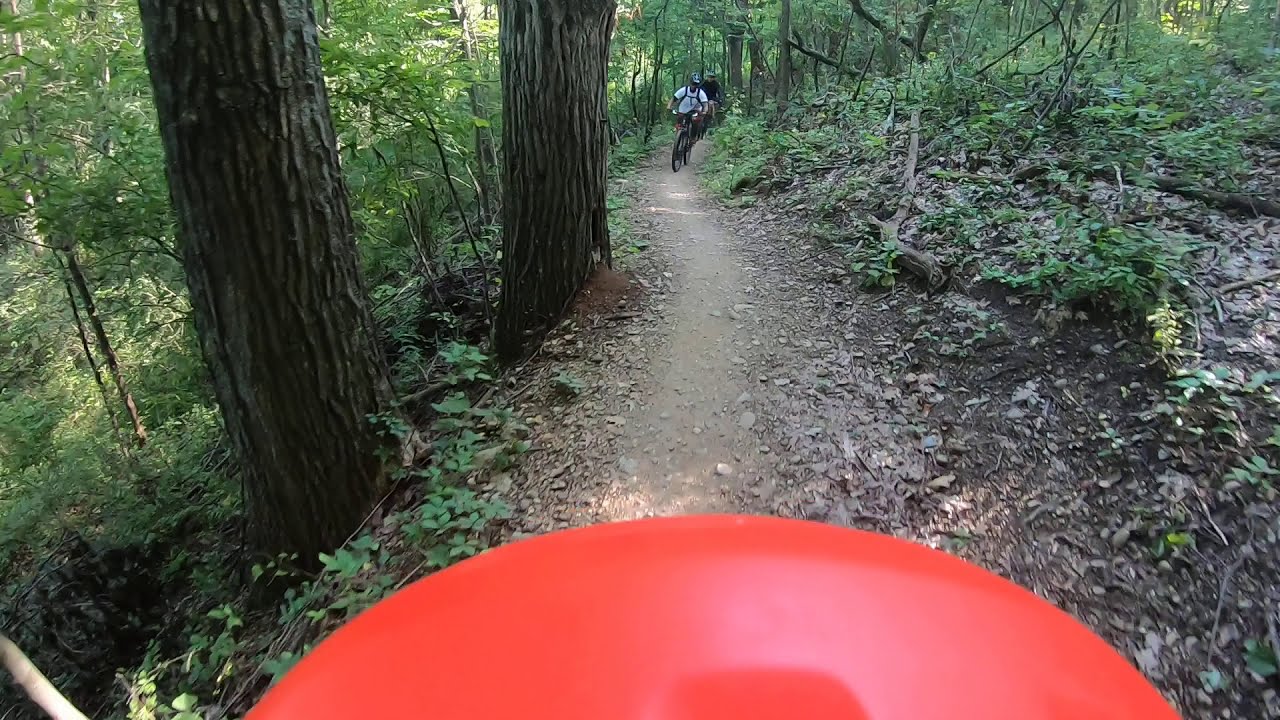In this detailed outdoor scene set deep within a forest, two large tree trunks dominate the left side of the image, surrounded by verdant greenery. A winding dirt path cuts through the middle of the scene, bordered by a small grassy hill on the right, scattered with branches. Toward the front of the image, a conspicuous half-circle of a red object, possibly the front of a motorcycle or a large balloon, stands out prominently. In the distance, two figures on bicycles are visible, headed towards the camera. One cyclist wears a helmet and a white t-shirt, the other in black, both appearing small against the lush backdrop of trees and dense foliage that envelops the path on all sides. The scene exudes the tranquility of a wooded area, with an overarching sense of green and brown hues, punctuated by the mysterious red object in the foreground.